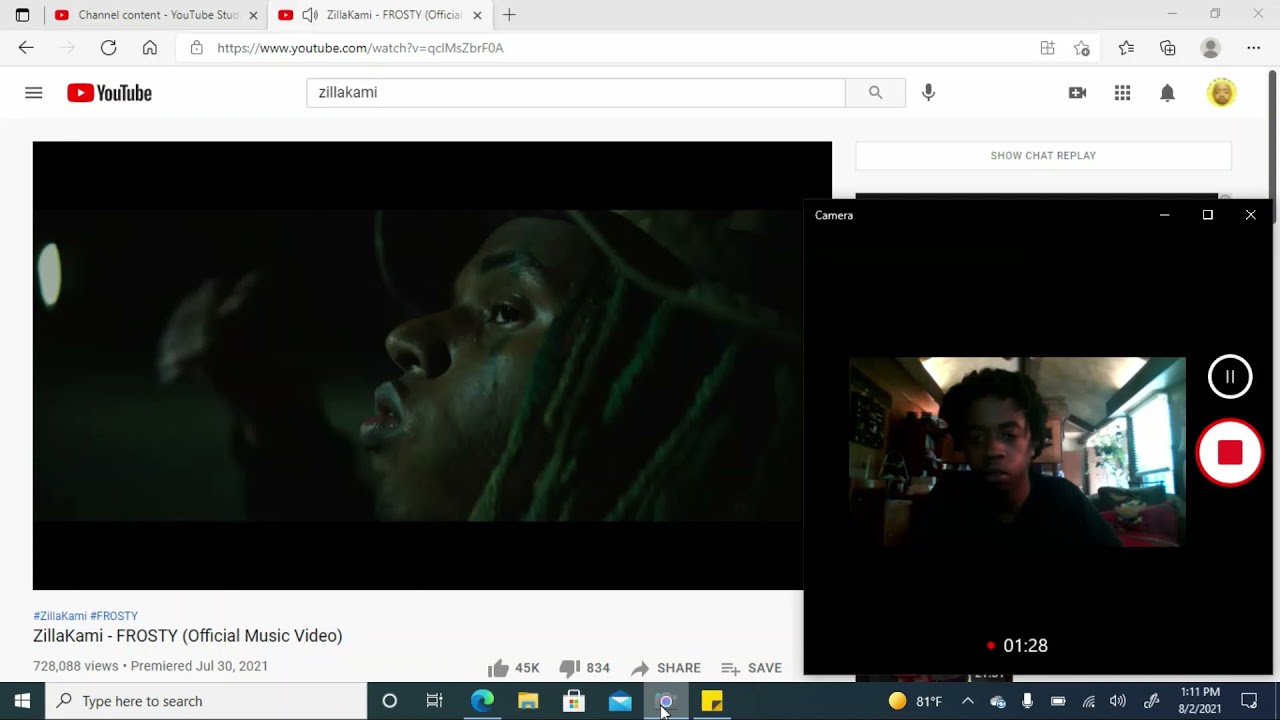A screen capture of a YouTube webpage displays the "Zillow Cammy - Frosty Official Music Video." The video player shows a frame featuring the side profile of an African individual's head. This person wears a cap over their dreadlocks and appears to be driving a car. The video is paused, making it unclear what the audio might be. Additionally, there is an inset image of another African individual, labeled "camera," suggesting a recording in progress. This person might be providing commentary or vlogging about the music video. The interface elements, such as the YouTube logo and video controls, are also visible, indicating this content is being viewed directly on the YouTube website.